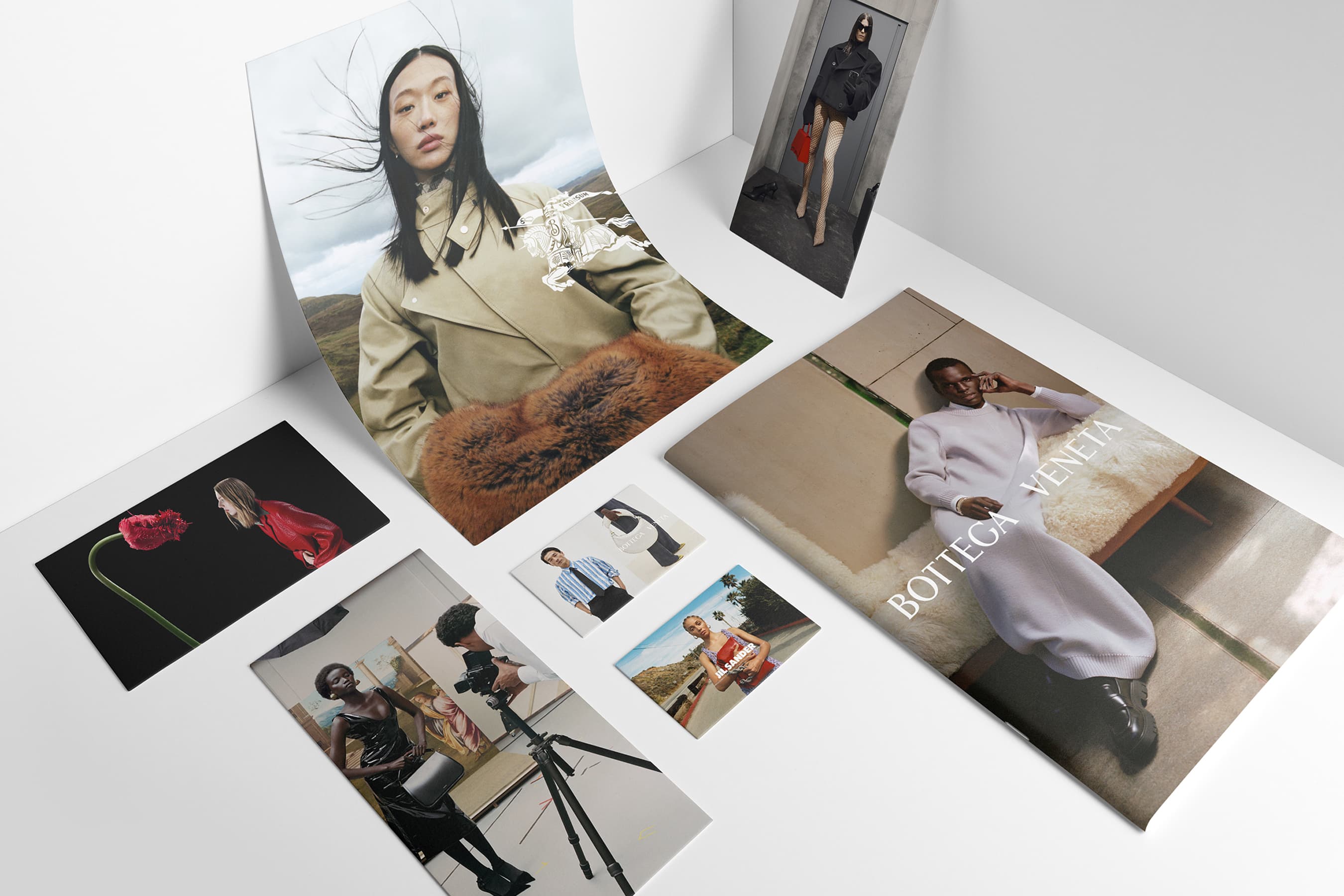The image captures a bird's-eye view of several color photographs scattered on a white table or possibly a white cubicle floor. The first photograph, positioned at the lower left-hand corner, depicts a woman gazing at an enormous red rose with a green stem. Below this is a photo of a photographer capturing a model in a black dress holding a purse. To the right, two smaller photographs are positioned vertically: the top one features a man in a blue and white shirt with a tie, while the bottom one shows a woman in an orange dress staring directly at the camera. Above these, leaning against a white wall, is a large photograph of an Asian woman in a tan coat with her hands in a brownish-red fur muff. Adjacent to this is a smaller, vertical photograph of a person standing, dressed in a black jacket that barely covers their hips. The final image at the bottom of the arrangement features an African American man lounging on a couch or cot, draped in a cream-colored fur throw, wearing all white. The photograph prominently displays the words "Bottega Veneta" in the center in white, capital text.